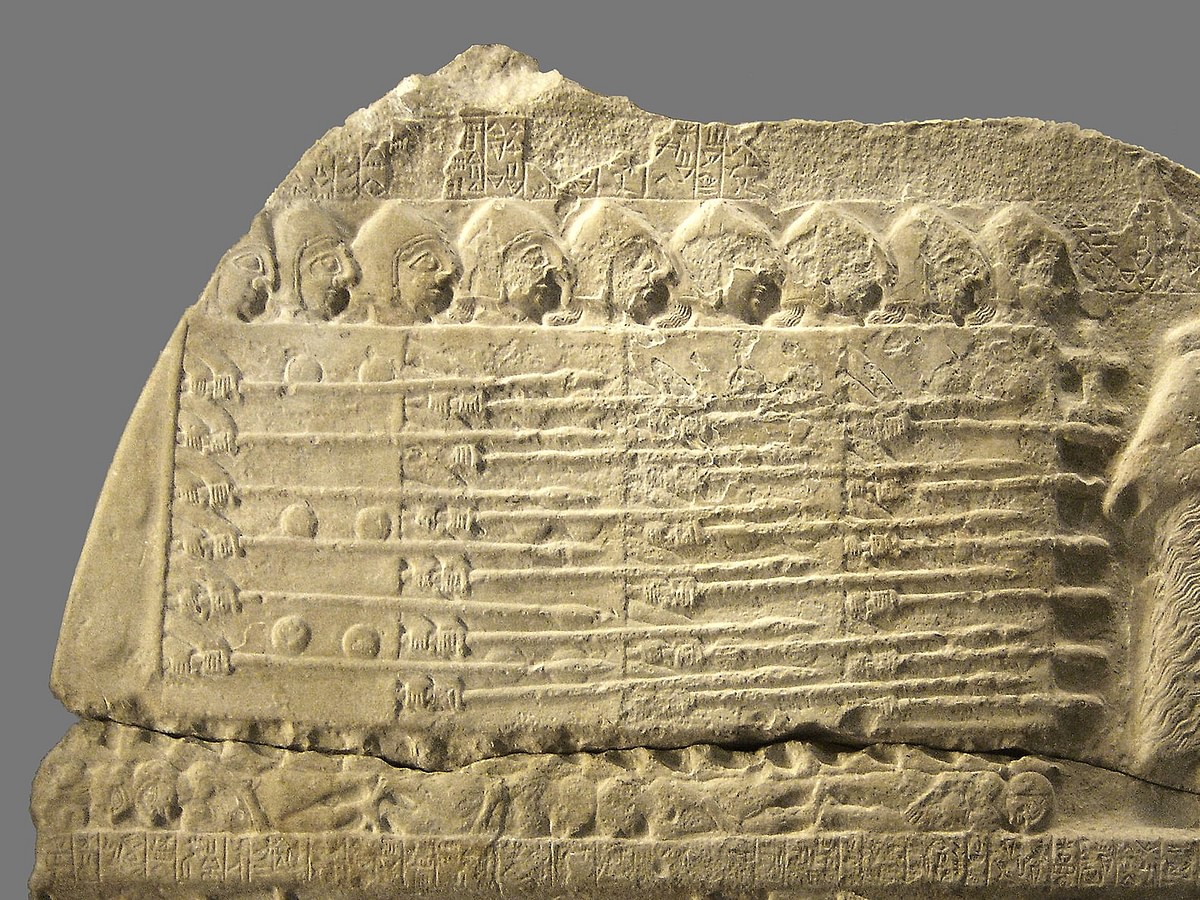The photograph showcases a close-up of an ancient stone engraving, taking up the majority of the image and set against a gray background. The light brown stone, worn and chipped over time, depicts a scene of soldiers marching from left to right. The soldiers are shown in profile, heads adorned with helmets and bodies shielded, suggesting a protective wall formation. The figures are holding what appear to be swords or spears, and their path is strewn with the bodies of fallen individuals. Intricate carvings, possibly cuneiform, decorate parts of the slab, though some sections are chipped and smoothed over. Above the soldiers' heads, partially chipped-off script adds a further layer of historical intrigue to this captivating artifact, presumably from an ancient Middle Eastern or Egyptian civilization.